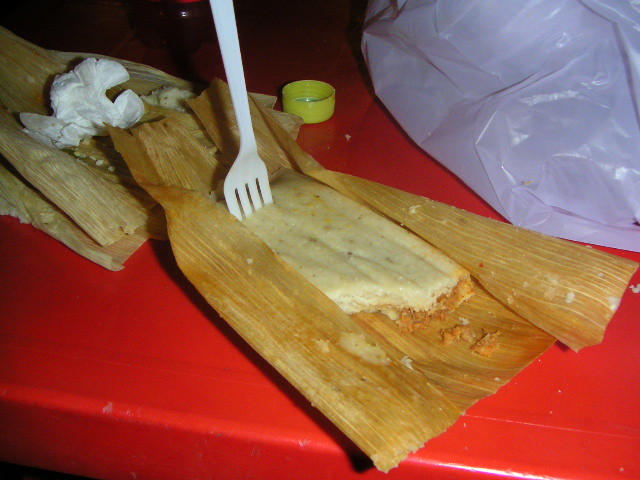A half-eaten tamale, wrapped partially in a yellow corn husk, sits prominently on a bright red plastic table. The tamale, made of a pale masa corn meal, has a white plastic fork stuck into its left-center portion, indicating a paused meal. Two discarded tamale husks and a white napkin lie to the upper left, suggesting this is the eater's third tamale. A small yellow plastic bottle cap sits just right of the fork. In the upper right corner of the scene, there is a crumpled white plastic bag that likely carried the tamales, highlighting an ongoing, yet unfinished dining experience. The vivid red table surface, possibly a bench or car trunk, adds a striking contrast to the earthy tones of the tamale and its husk.